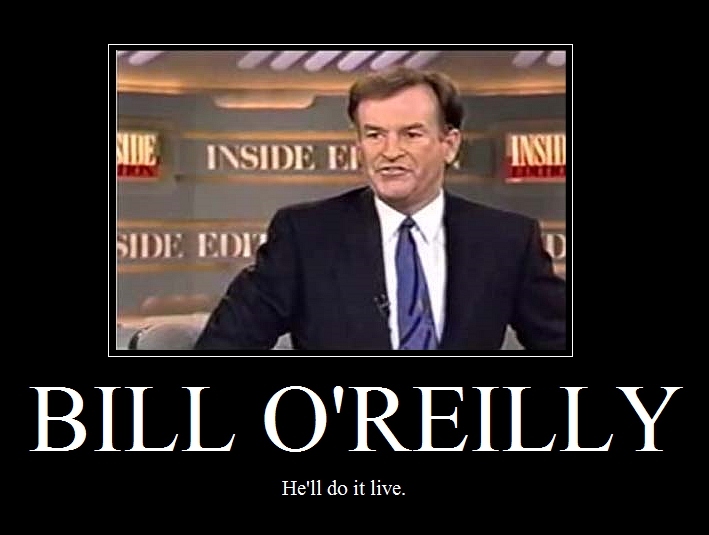This photograph features a younger Bill O'Reilly during his tenure as an anchor on "Inside Edition." The image is framed by a thick black border, with O'Reilly's name prominently displayed in large white capital letters at the bottom. Below his name, in smaller print, it reads, "He'll do it live." O'Reilly is dressed in a black suit, blue tie, and white shirt, sporting short brown hair. His facial expression is a noticeable scowl or grimace. The studio background of "Inside Edition" is visible behind him, adorned with differing stripes of lighting and text. The photograph has a slightly blurry quality.